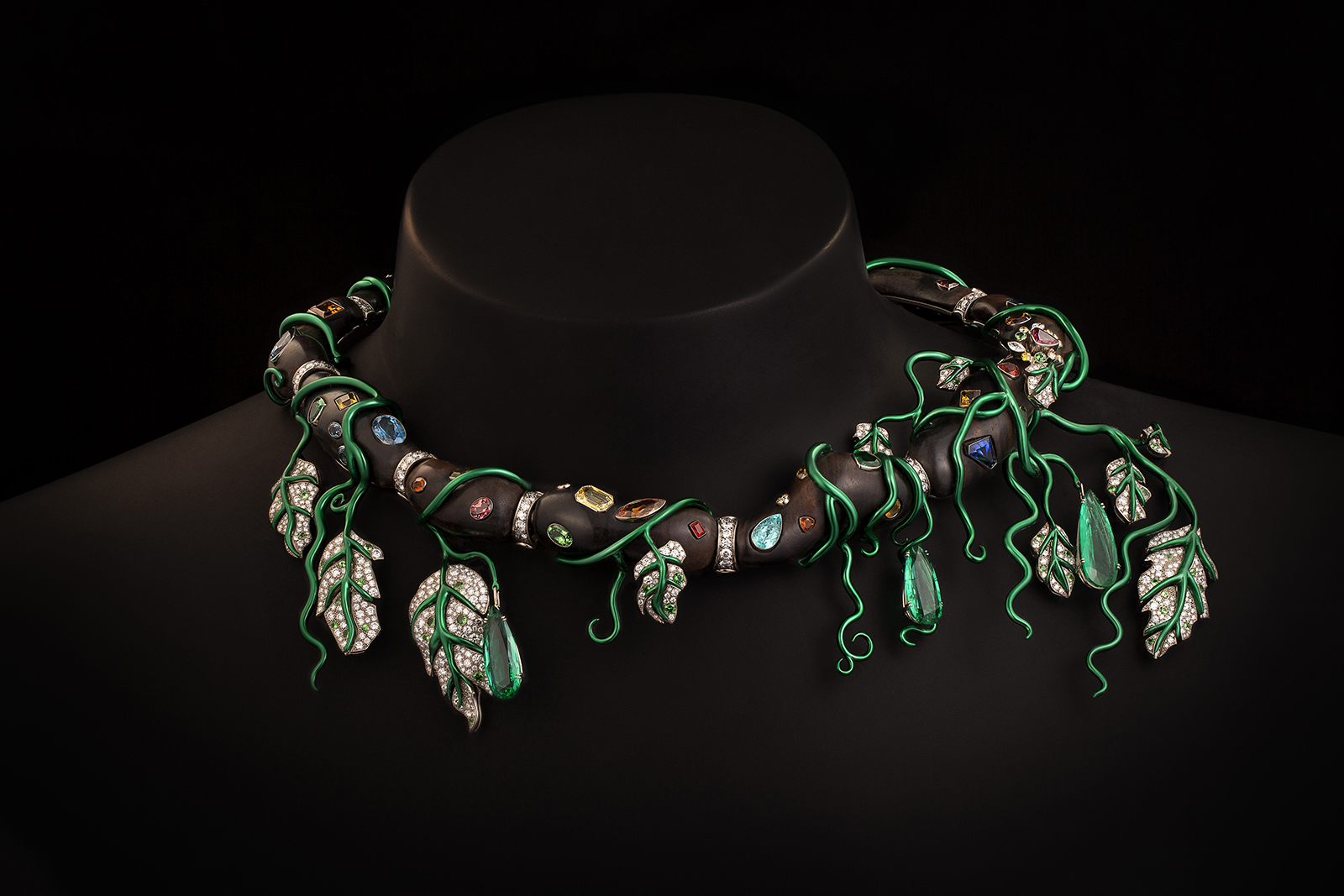This image showcases a close-up photograph against a black background, focusing on a headless black mannequin with a smooth, circular neck. The mannequin features a striking necklace, intricately designed with various multicolored gemstones including blue, yellow, green, pink, teal, and darker blue stones. The black necklace is adorned with green vines and leaves, some of which appear to be encrusted with diamonds or white-colored gems. The detailed craftsmanship of the necklace, which may include elements resembling both metal and organic forms, stands out vividly against the mannequin's dark surface.